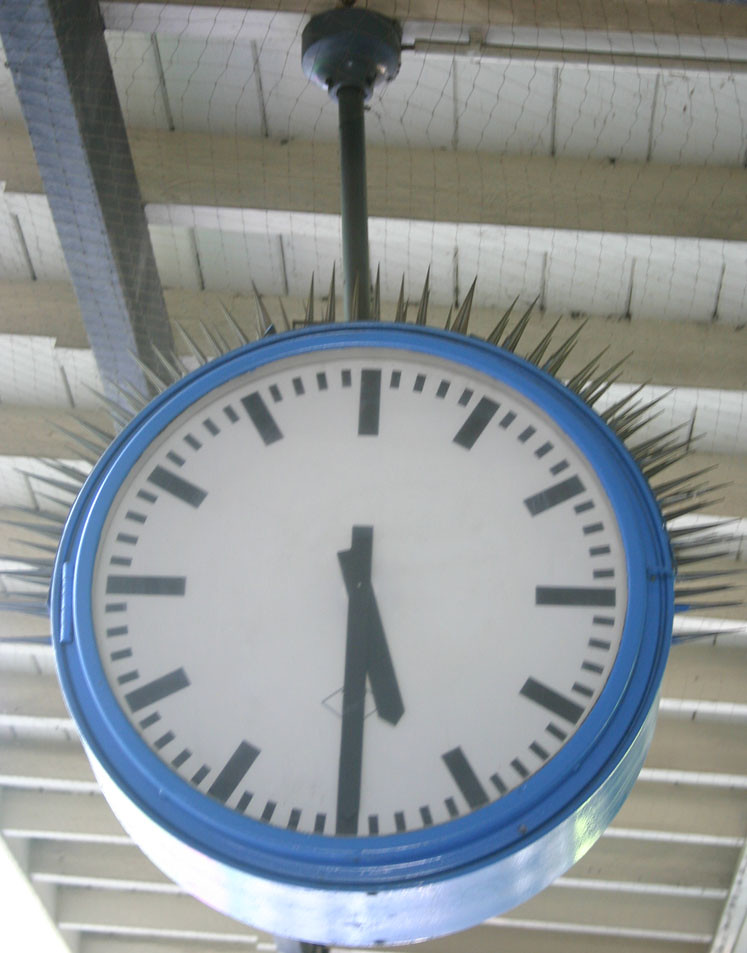This image captures a rustic, unfinished ceiling featuring horizontal wooden beams that extend the entire length of the frame. The wood possesses a natural light hue, adding a warm, earthy tone to the setting. Suspended from the ceiling is an eye-catching, large clock. Its hardware, a stark and sturdy black, contrasts sharply with the vibrant blue clock body. The face of the clock is white, adorned with minimalist black lines marking the hours and minutes without any numeric indicators, providing a sleek and modern aesthetic. It displays the time as 5:35. Adding a unique and somewhat edgy element, the top half of the clock is adorned with silver spikes, radiating outwards and giving the appearance of dangerous, pointed rays.